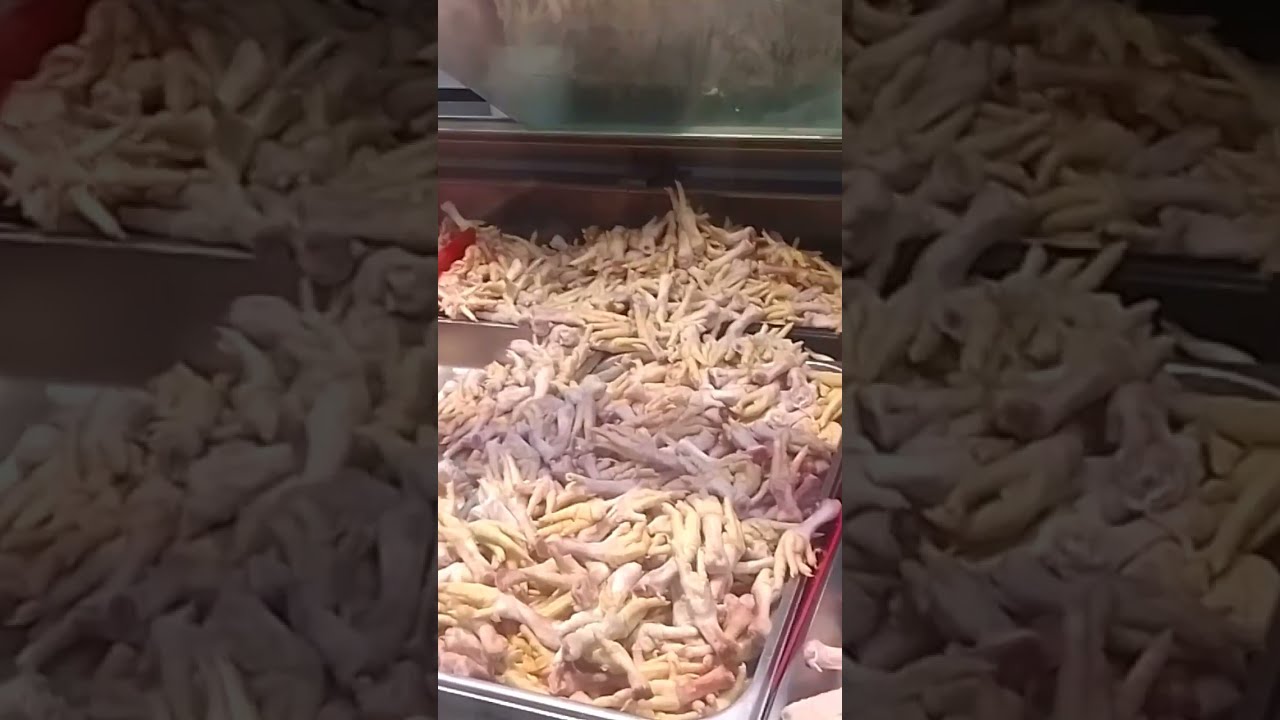This image shows a horizontal rectangular composition divided into three equal vertical sections. The middle section is brightly illuminated and in color, clearly showcasing a deli counter. In it, a prominent horizontal pan filled with what appear to be chicken feet is visible, positioned beneath a small window. The left and right sections are significantly darker and somewhat obscured, depicting silver trays similar to those in the center. On the left, there is a vertical tray stacked above another, both containing a mass of chicken feet. The right section mirrors this arrangement with trays positioned similarly, displaying what appear to be chicken feet spilling out and filling the trays. The overall scene is somewhat disturbing due to the contents, but it seems to represent preparations for the items to be served as food. The framing and composition suggest a deliberate focus on the central lit section, contrasting with the shadowed peripheries.